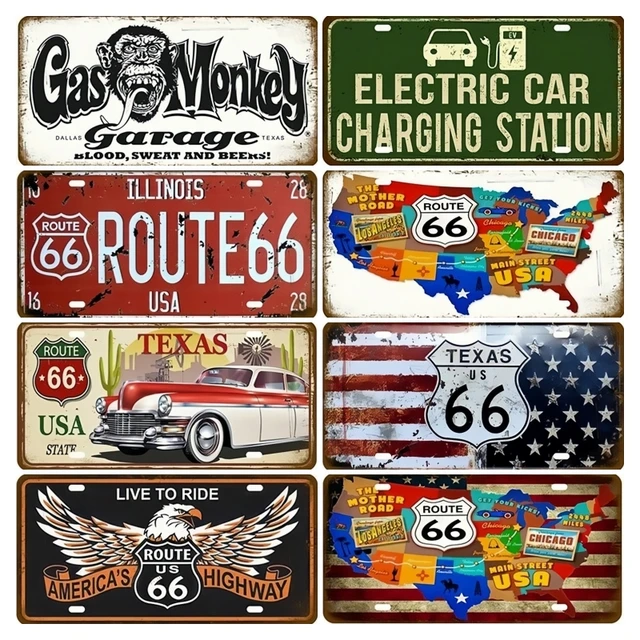This is a collection of eight decorative license plates, each designed to mimic real car plates but focused on various themes, with a strong emphasis on Route 66. They are organized in two rows of four. The top row features the following plates: The first displays the logo and a chimp face from Gas Monkey Garage; the second has a green background and says "Electric Car Charging Station"; the third is a weathered red plate with white lettering from Illinois' Route 66, USA; and the fourth shows a colorful US map with the Route 66 logo. The bottom row includes: a plate celebrating Route 66 in Texas, complete with a vintage car, windmill, and cactus; another plate with an American flag background and the Route 66 highway sign; a Harley-Davidson-themed plate stating "Live to Ride" with an eagle logo and the words "America's Highway, Route 66"; and finally, another plate similar to the colorful US map one, but also featuring the American flag as the background. Many of these plates show signs of rust and aging, adding to their vintage charm.